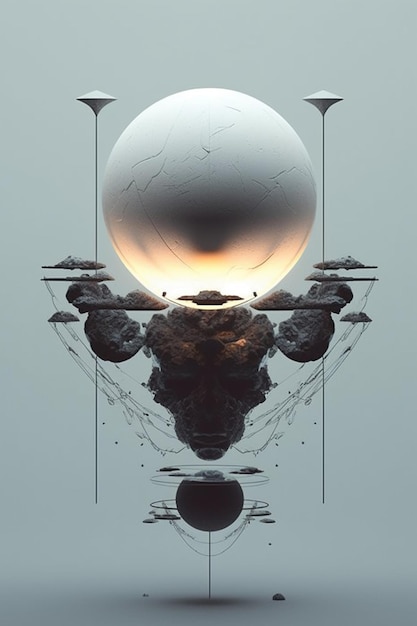The image appears to depict an abstract 3D art piece with a light blue-gray background. Central to the composition is a large, white sphere with a matte finish, illuminated from below, highlighting its surface and some distinct cracks. Beneath this glowing white orb is a symmetrical arrangement of black volcanic rocks, mimicking a semicircular formation. Among these rocks, a prominent piece stands out, resembling a tribal mask or a human head, complete with discernible eyes, mouth, and nose.

Flanking the white sphere are two small diamond shapes, each perched atop slender black lines, mirroring each other on the left and right sides. Below the volcanic rocks rests a smaller black sphere, intersected by yet another black line extending towards the ground, which casts a shadow. Subtly incorporated into the scene are cloud-shaped formations crafted from the same dark material, enhancing the abstract and harmonious nature of the artwork, though not all elements achieve perfect symmetry. A slight disparity is observable in the ground rocks, with the right side bearing a larger rock compared to the one on the left.